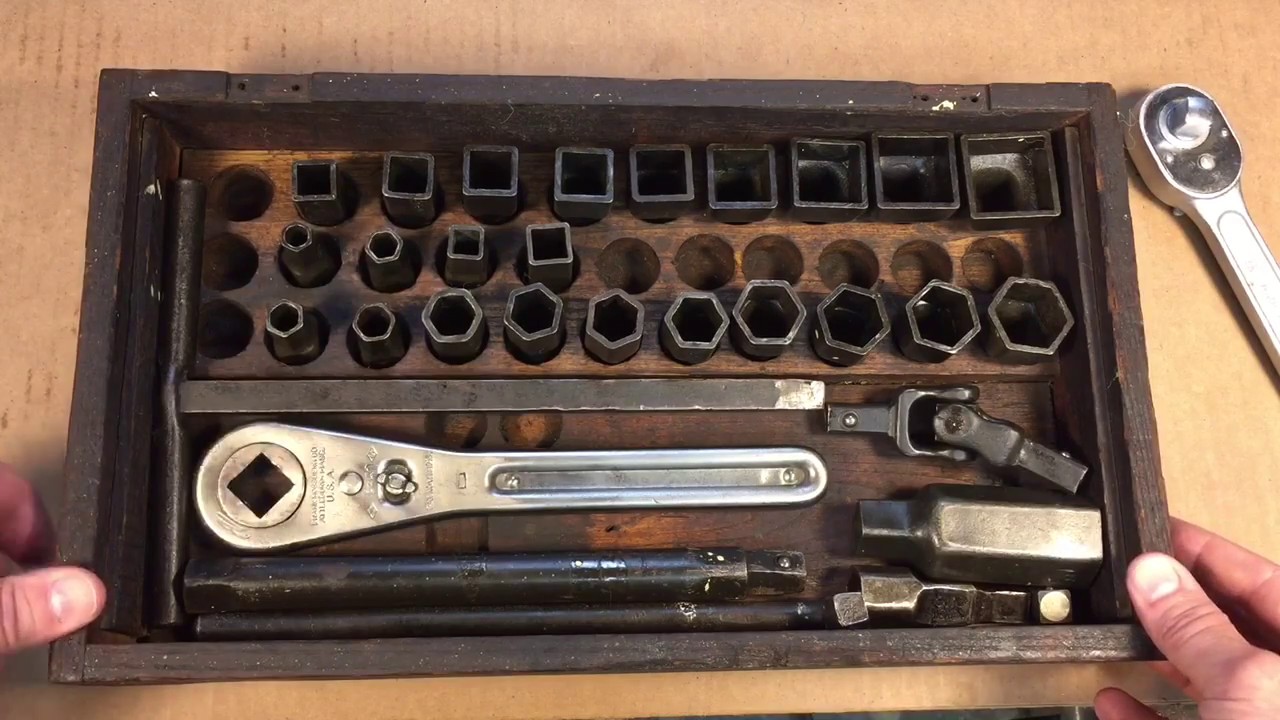The image is a color photograph showcasing an old-fashioned tool kit held by a person's thumbs visible in the bottom left and right corners. The rectangular tray, possibly made of wood or metal, and laid on a light brown, cardboard-like surface, is divided into multiple sections. The upper section of the tray features three rows of various sized bits, with some slots empty, indicating missing pieces. The first row contains numerous square metallic objects, while the second row holds four items—two circular and two square. The third row comprises round and octagonal pieces. The lower section of the tray houses metal tools, including wrenches and pliers, designed to fit the corresponding bits above. The background and the tray's contents suggest meticulous organization despite some missing components.